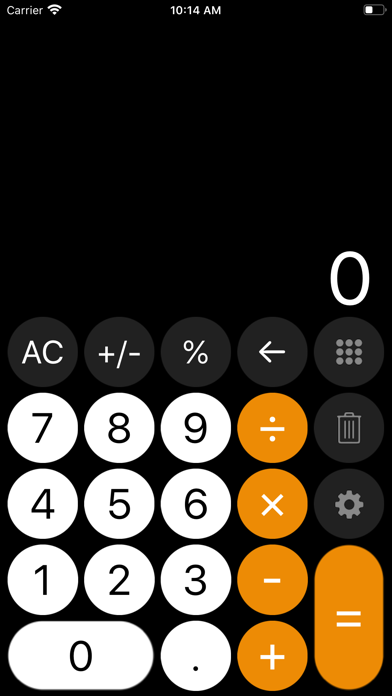The image is a close-up screenshot of a smartphone displaying its calculator app. At the top left corner, the screen shows the carrier name and a Wi-Fi icon indicating a strong connection. The time reads 10:14 AM at the center, and the battery icon on the top right indicates roughly 25% charge remaining.

Dominating the screen is a traditional calculator interface. The upper section of the calculator is relatively simple, unchanged from older designs. On the left side, a black circular button labeled "AC" is visible, followed by buttons for "±", "%", and a back arrow arranged in a row. The number pad is white, showing digits arranged in a standard format from 1 to 9, with 0 located in a larger circle at the bottom of the pad. A dot button next to zero prompts the user to input decimal points.

On the right side of the calculator interface, there are four orange circular buttons for arithmetic operations: division (÷), multiplication (×), subtraction (−), and addition (+). The minimalist, functional design of the calculator app emphasizes ease of use, similar to earlier versions of digital calculators.